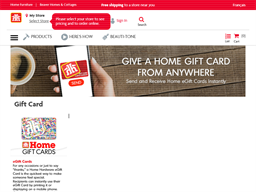A website advertisement showcases the convenience of sending home gift cards from anywhere. The banner features a cozy photograph of a steaming mug of coffee and a woman holding a smartphone in her right hand, presumably displaying the app used to send these gift cards. To the right of this image, bold text announces, "Give a Home Gift Card from Anywhere." Above this text, albeit in very small and somewhat unreadable font, are options like "hamburger," "products," and a search icon, all enclosed within a red border. Below the main photograph, the text "Gift Card" appears prominently, reiterating the theme of the webpage. The webpage promotes the ease of using a mobile app to select and send gift cards, highlighting its user-friendly nature despite the small, difficult-to-read text details.